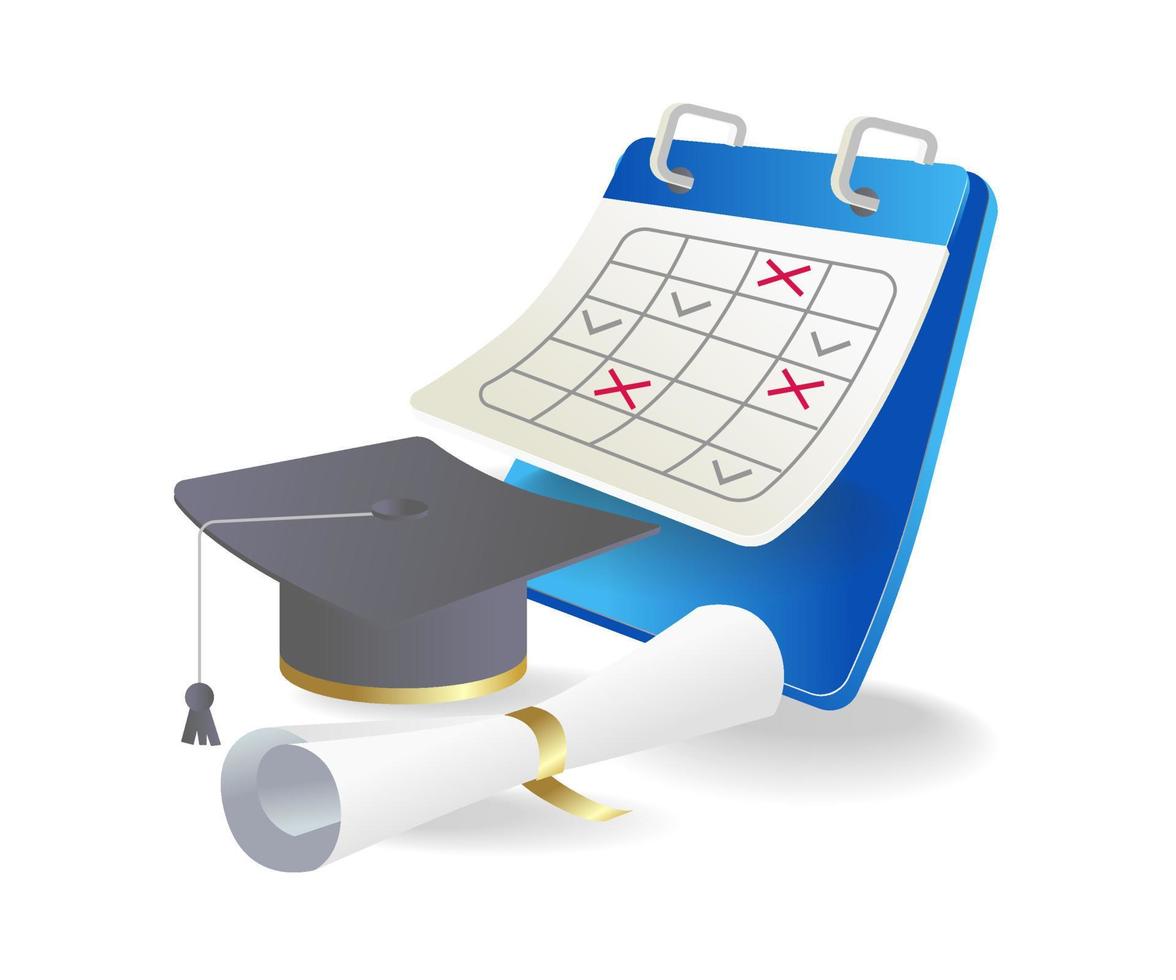This graphic features a blue spiral pad designed to resemble a calendar or clipboard. The paper on the pad displays a grid with four columns and five rows, where some squares contain red X's and others gray check marks, seemingly placed at random. Positioned in front of this calendar-like structure are a gray graduation cap with a gold band around the rim, complete with a tassel, and a coiled, rolled-up diploma tied with a gold ribbon. The image is set against a completely white background, with shadows cast by the objects, suggesting themes related to academic milestones or graduation preparation.